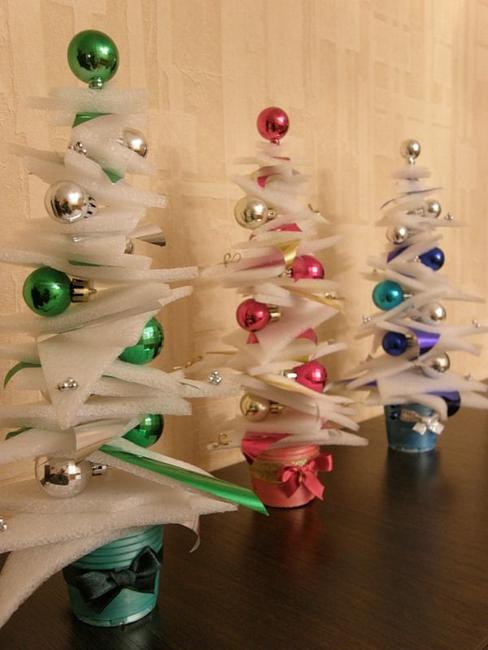This captivating image showcases three handcrafted Christmas tree decorations, each crafted from white styrofoam and adorned with colorful ornaments. The scene is set against a textured beige wall with a subtle wood grain pattern. The floor has a lustrous finish, displaying heavily polished oak boards that create a faint reflection.

The three tree sculptures are placed on a dark brown wooden table, arranged diagonally from front left to back right. Each tree sits in a small, vividly colored pot with matching ribbon bows. The frontmost tree rests in a green pot with a dark green ribbon, the middle tree is in a red pot with a pink ribbon, and the furthest tree is in a blue pot with a gold ribbon. The triangular foam pieces that constitute the trees are stacked with the widest parts at the bottom, narrowing towards the top, and are randomly oriented to form an abstract yet recognizable tree shape.

The green tree is decorated predominantly with green and silver baubles, including a prominent green bauble at its top. It also features interwoven green ribbon throughout its foam layers. The middle tree in the red pot (occasionally described as pink) showcases pink and silver baubles, with a pink bauble crowning the top, and includes some ribbon detailing. The blue tree at the back is adorned with blue, turquoise, and purple baubles, accented by gold baubles, and it is topped with a gold bauble. This tree also features a combination of blue and purple ribbons interlaced among its foam triangles.

Despite varied descriptions of the pot colors and ribbons, this unique display resonates with a festive, handcrafted charm, merging traditional Christmas elements with a modern, artistic twist.